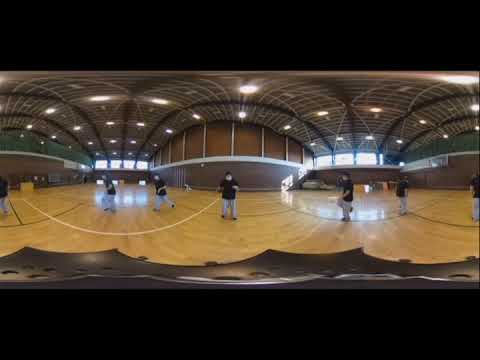The image is a blurred and compressed fisheye lens photograph, likely taken indoors in a gymnasium. This panoramic shot creates a wavy, rounded appearance, especially in the middle and edges of the picture. The gymnasium features a polished light brown wooden floor with various black and white markings. It has darker brown walls with brown curtains covering some of the windows, while other windows are open and allow sunlight to stream through, suggesting it's afternoon. The ceiling is brown with darker beams and numerous light bulbs. The gym has four large windows on one wall and additional windows on the right side, creating a well-lit environment. On the court, there are six or seven individuals, presumably children, wearing matching black short-sleeved shirts, gray pants, and occasionally white face masks. Despite the image's blurred quality, details like the green and brown walls and the heavy shine on the wooden floor are discernible. The photograph also includes some black header and footer bands, possibly indicating it's a screenshot from a video.